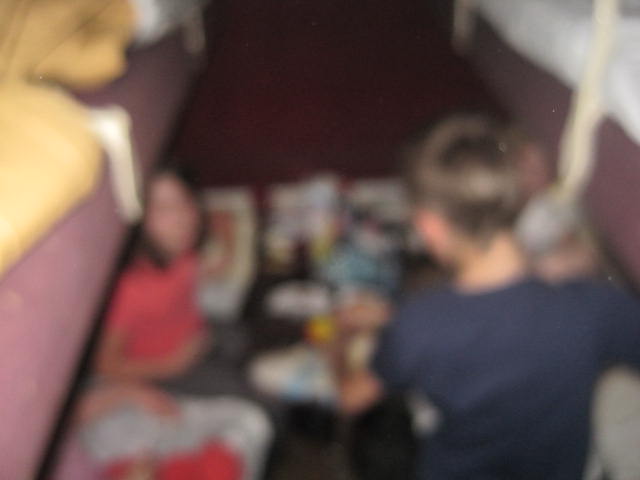This photograph, although very blurry, captures a poignant moment between two children. The child in the center has short brown hair and is wearing a navy blue t-shirt, while the child on the left sports longer brown hair and is dressed in a pink t-shirt. To the left of the image, there is a rusty red couch with distinct yellow seat cushions. The scene is set against a dark-colored floor, scattered with various colorful objects - white, blue, red, and yellow - resembling the aftermath of a Halloween candy display. On the right side of the image, a bed with a matching rusty red frame and white sheets adds to the homely ambiance. The blur indicates that the photo was taken with a shaky hand, adding an element of motion and spontaneity to the captured moment.